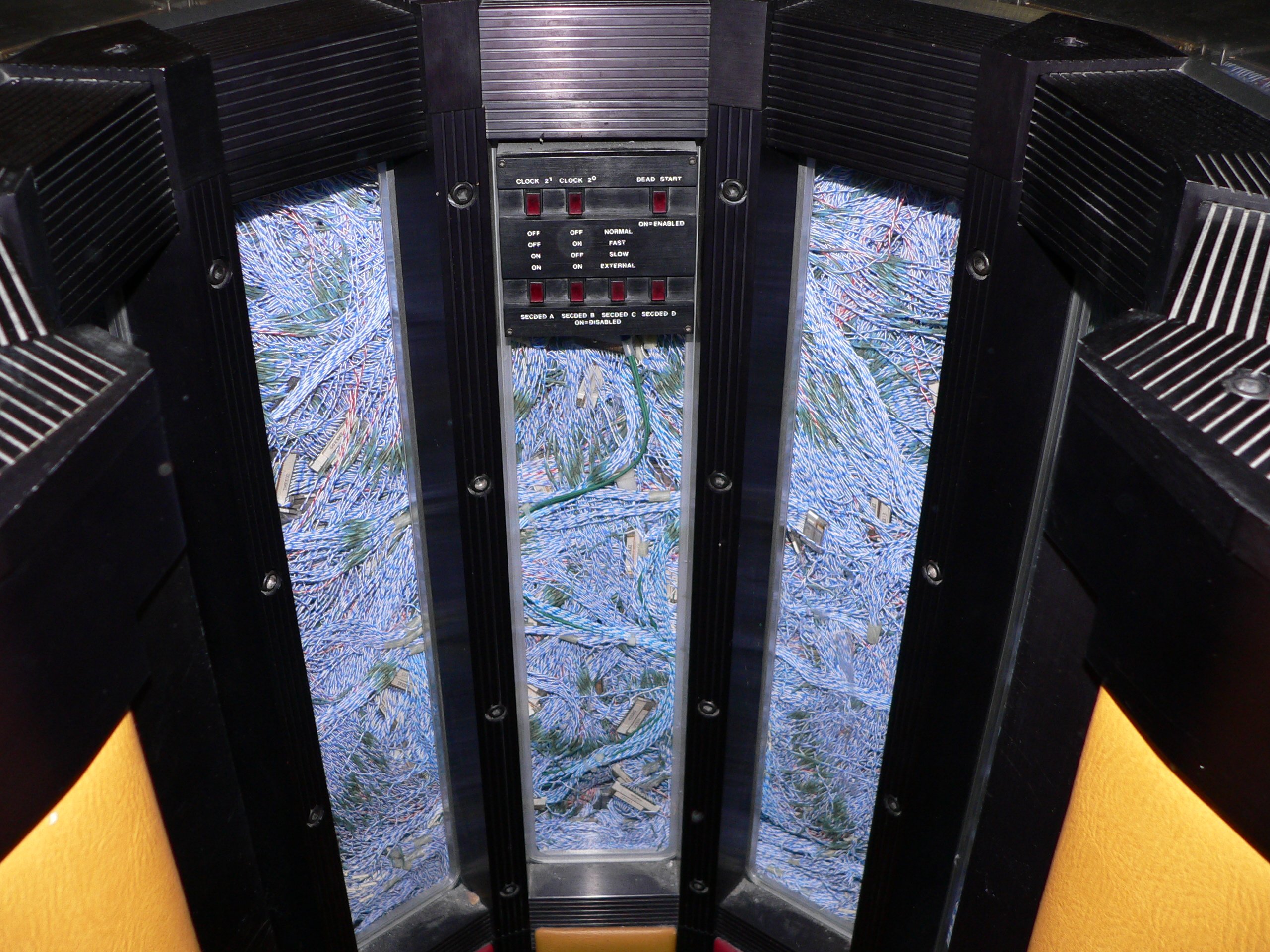The image features a predominantly black machine, meticulously detailed in composition. The various components of the machine, including screws, are uniformly black, creating a sleek and cohesive appearance. Central to the machine are three glass sections, with the middle glass being slightly shorter than the two flanking it on the right and left. These glass sections house numerous cable codes, which are visible and clustered behind them. The cables come in various colors, predominantly blue and white, with occasional green and red hues. Each cable is equipped with white connectors, adding a stark contrast against the darker background.

At the base of the machine, on both the bottom left and right, there are yellow accents that add a vibrant touch to the design. Above the central glass panel, red text is prominently displayed, listing various operational settings and statuses in a technical and precise format: "clock 2 1, clock 2 0, dead start, on enable, normal, easy, slow, external, off on, off on, second A, second B, second C, second D, on disabled." This text adds an element of functionality and technical detail, suggesting the machine's complex operational capabilities.